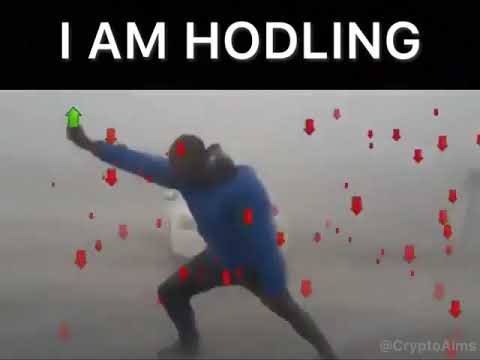The image is a blurry and somewhat indistinct meme, likely intended for a cryptocurrency audience, featuring a central figure who is difficult to make out clearly but appears to be a man wearing a blue long-sleeved shirt and black pants. His head is obscured by a black object, possibly a ski mask. The man is depicted in a dynamic pose with his legs spread apart—his right knee bent forward and his left leg stretched out behind him. His right arm is raised above shoulder level, holding a green arrow pointing upward, while his left arm is down by his thigh. The background is predominantly white or light gray, punctuated by numerous red arrows pointing downward. At the top of the image, a black rectangular strip contains the phrase "I am HODLING" in bold white letters, referencing the cryptocurrency slang for "Hold On for Dear Life." In the lower right corner, there is the white text "at Crypto Ames," attributing the meme.